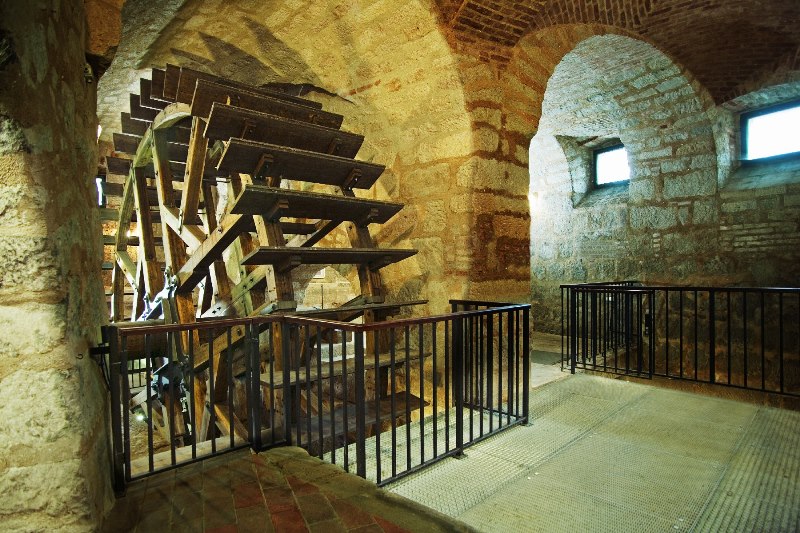The photo captures the interior of a vintage brick building, now presumably a tourist attraction. Central to the image is a large wooden waterwheel, historically used for water-powered machinery before the advent of electricity. This waterwheel, crafted from wooden boards and studs, is set into motion by a flowing water feature. Surrounding the waterwheel is a protective wrought iron fence, safeguarding visitors from potential harm. The building's architecture includes curved archways and a concrete viewing area, emphasizing its historical significance. Sunlight streams through two upper-right windows, illuminating the brick walls with a warm orange glow, highlighting the detailed craftsmanship of this bygone era.